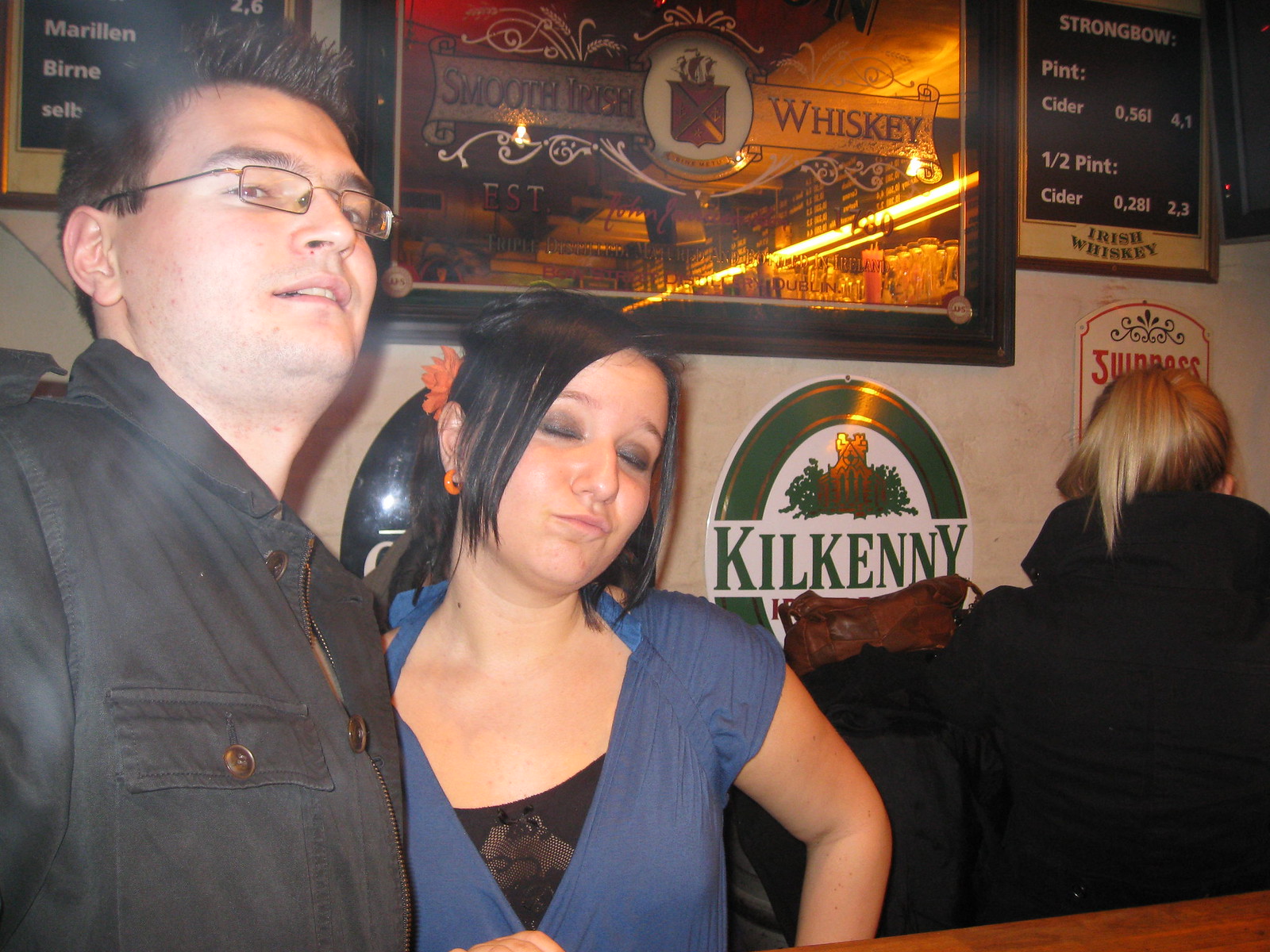In a bustling Irish-themed pub, a young Caucasian couple with dark hair stands out in the foreground. The woman, wearing a black shirt under a blue blouse, has heavy dark eyeshadow and her eyes closed, possibly indicating she's drunk. Her black hair is accessorized with an orange flower and matching earring. Next to her, the man sports short dark hair, wire-frame glasses, and a black shirt with brown buttons. His gaze is directed upwards. Behind them, a blonde woman with her back to the camera is slightly visible. The walls are adorned with numerous pub signs and mirrors, emphasizing Irish heritage with labels such as "Kilkenny," "Smooth Irish Whiskey," and "Strongbow." A black sign with intricate leafy designs, another sign mentioning “Marilyn, Bernie, Selb, 2.6”, and multiple listings like "Pint Cider," "Half Pint Cider" in white on black backgrounds add to the pub's authentic atmosphere. The detailed decorations and dim ambiance reflect the couple's immersive, albeit inebriated, experience.